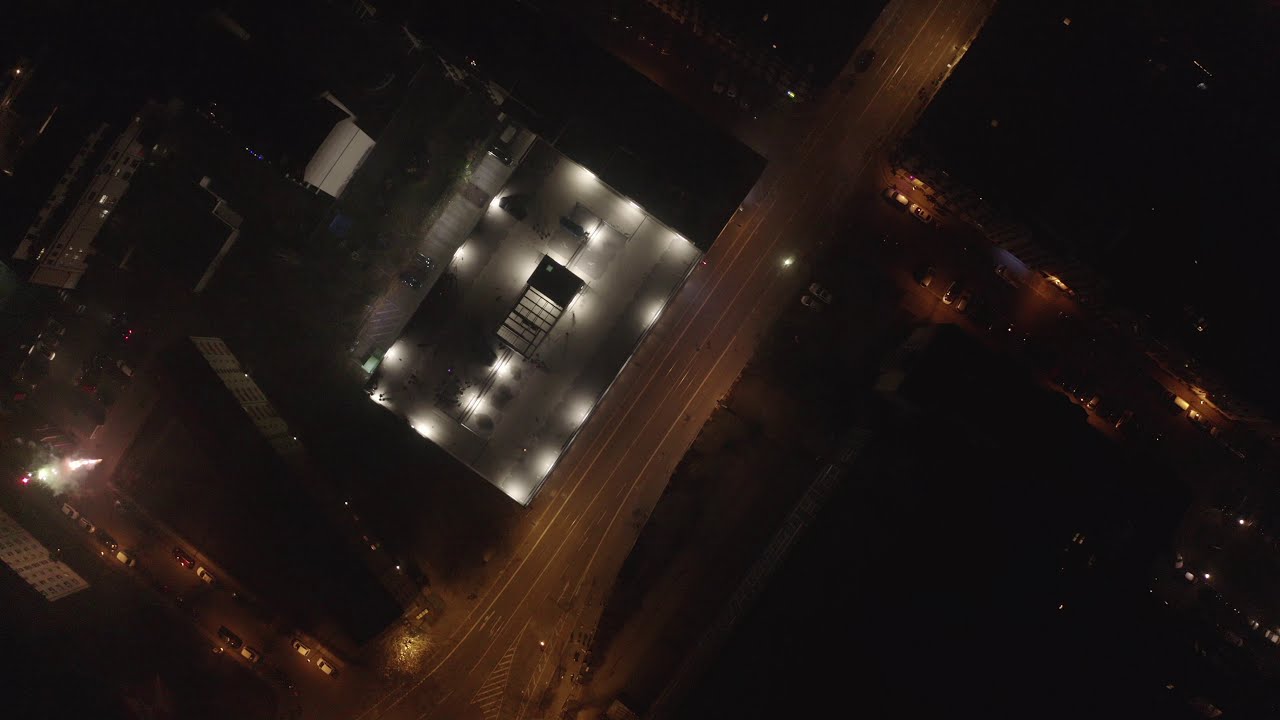This aerial nighttime photograph showcases an urban landscape from a bird’s-eye perspective. Dominating the composition is a diagonally positioned multi-lane road that runs from the bottom left to the upper right, intersected near the top right by another four-lane street, which stretches from the middle left to the bottom right. Both roads are illuminated with warm, amber-hued streetlights, casting a dim glow over the scene. The roads are relatively sparse with parked cars scattered throughout. On the left side of the main road, a well-lit building stands out prominently with bright white lights atop its roof, in contrast to the other structures, which are dimly lit with yellow lights emanating from their sides. The majority of the building rooftops are shrouded in darkness, presenting nearly oppressive black surfaces that hint at the depth of the night. The setting is devoid of any text or visible signage, and the color palette consists of subdued tones of white, yellow, orange, black, gray, silver, and tan, underscoring the nocturnal atmosphere.